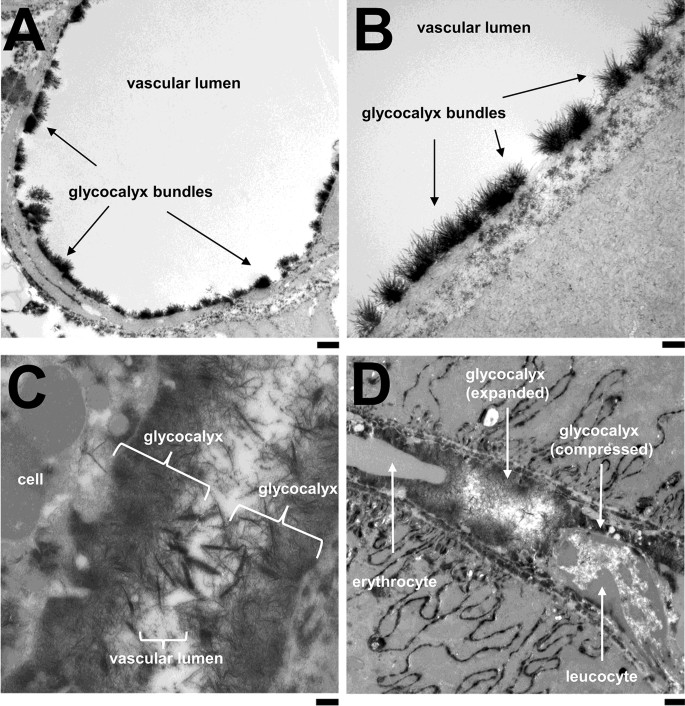The image is a composite of four high-contrast black and white microscope images arranged in a square grid, each labeled with letters: A at the top left, B at the top right, C at the bottom left, and D at the bottom right. Each image is meticulously annotated with arrows and challenging biological terms. Images A and B are labeled "vascular lumen" and feature glycocalyx bundles, likely at different magnifications. Image C is marked with "glycocalyx" and shows cell structures without a given scale. Image D is labeled with "glycocalyx expanded," "glycocalyx compressed," "erythrocyte," and "leukocyte." The detailed annotations and clear visibility make it conducive for educational purposes, such as a biology class focused on cellular and nanoparticle analysis.